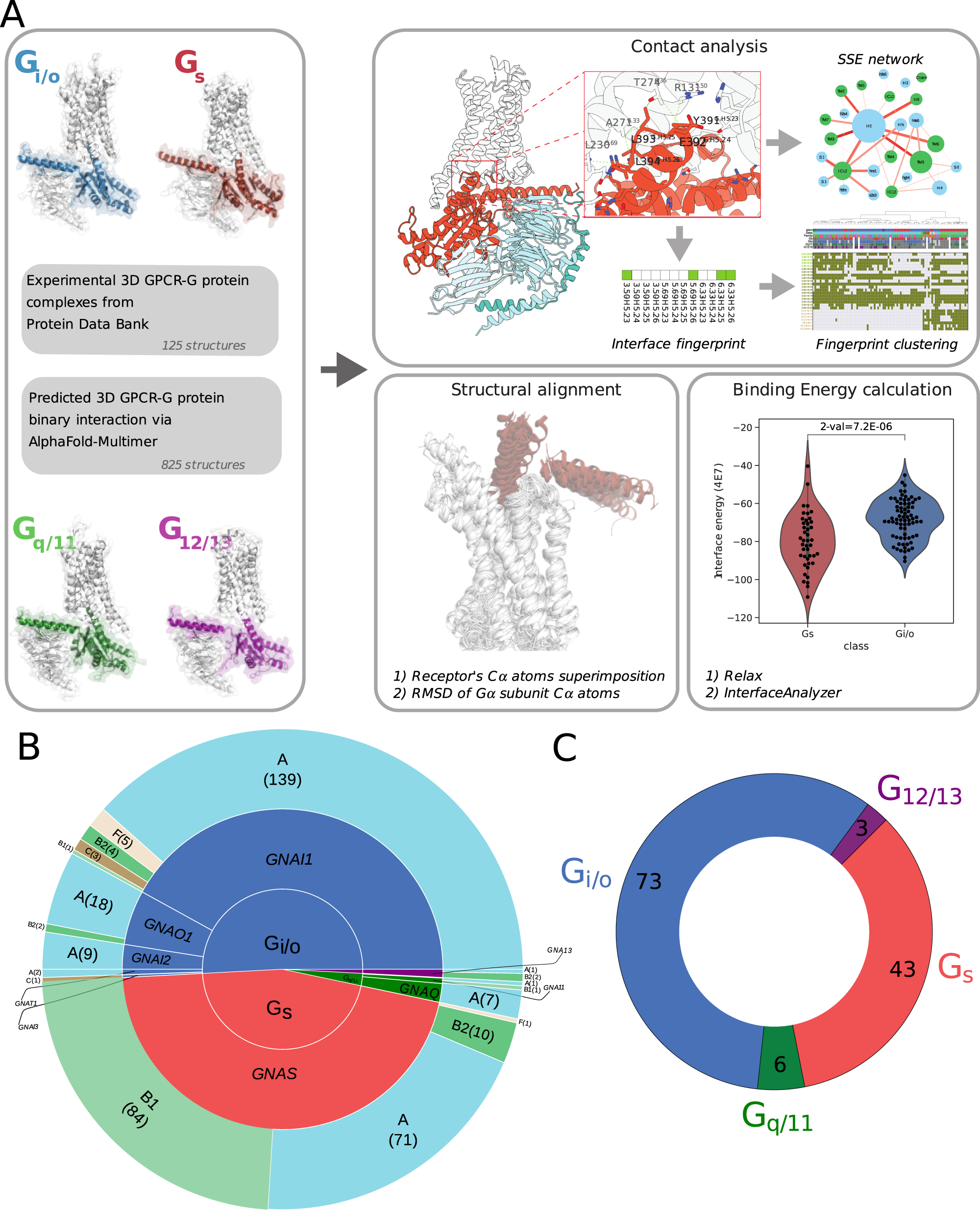The image is a detailed medical or scientific diagram, likely related to biotechnology or molecular biology. It is divided into three main sections labeled A, B, and C. At the top of the image in Part A, there is a vertical rectangle, two squares, and a horizontal rectangle. This section also features coil-like structures, which likely represent enzymes or protein structures. Each of these shapes contains text in gray text boxes with small black text, outlining concepts such as contact analysis, structural alignment, and binding energy calculation.

Parts B and C are represented by two circular graphs at the bottom of the image. The graph in Part B consists of concentric circles, while the graph in Part C is donut-shaped. These multicolored graphs, featuring colors like blue, red, and green, include black text with numbers and letters, potentially depicting various analytical data.

Overall, the diagram illustrates intricate details of a biological function on a microscopic level, incorporating atomic and energetic information, proteins, chemical reactions, and detailed analytical metrics.